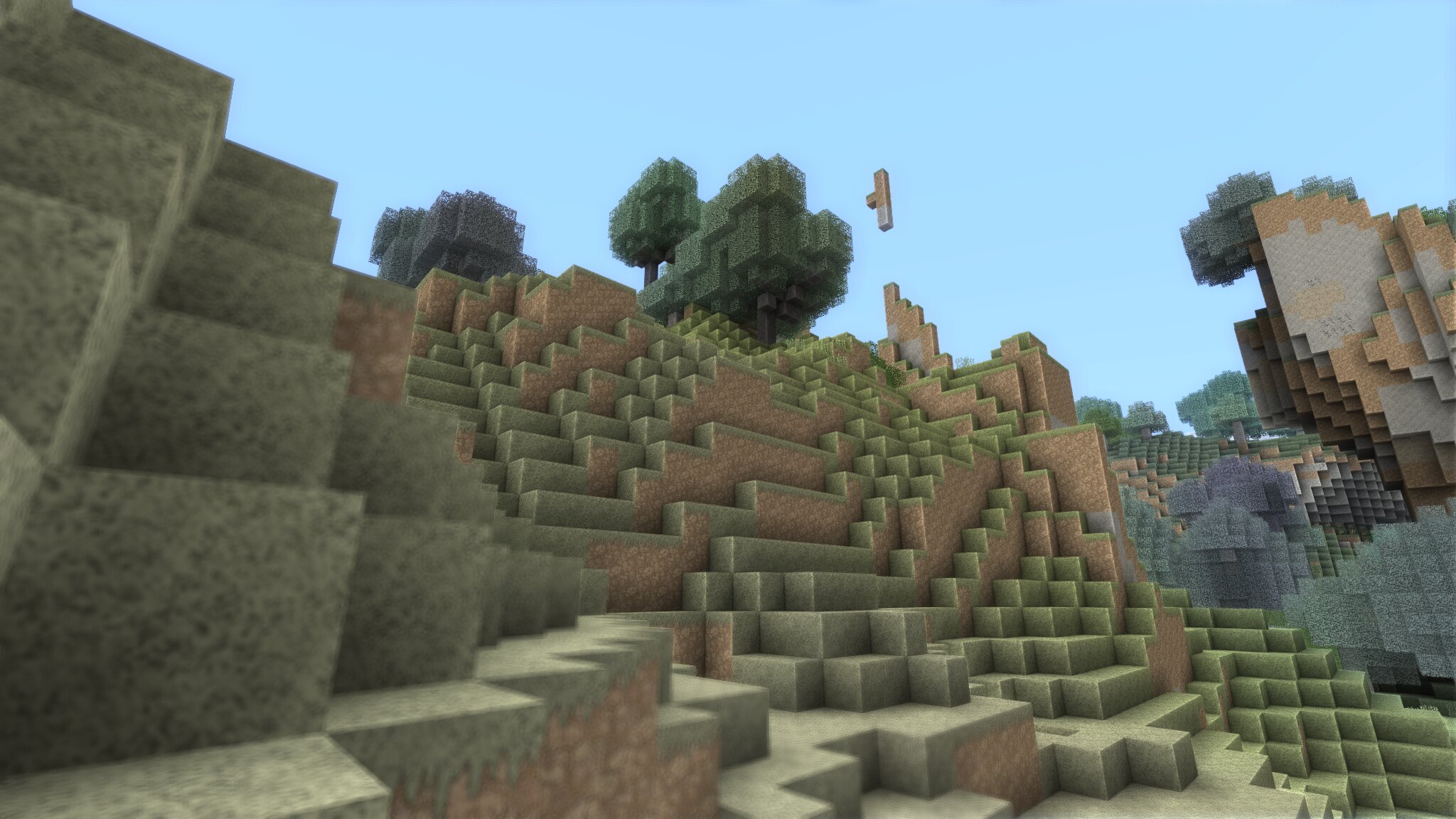The image appears to be a still from the video game Minecraft, showcasing a computer-generated outdoor scene. The background reveals a clear blue sky devoid of any clouds. In the foreground, the terrain is depicted with sloped areas composed of square blocks featuring muted shades of green and brown, indicating grass on the surface and dirt or soil beneath. Further back, there are clusters of dark green trees adding depth to the scene. On the right side of the image, several grayish blocks suggest the presence of stone. A small segment, consisting of a couple of blocks, seems to be suspended in midair as though it is in the process of being placed.